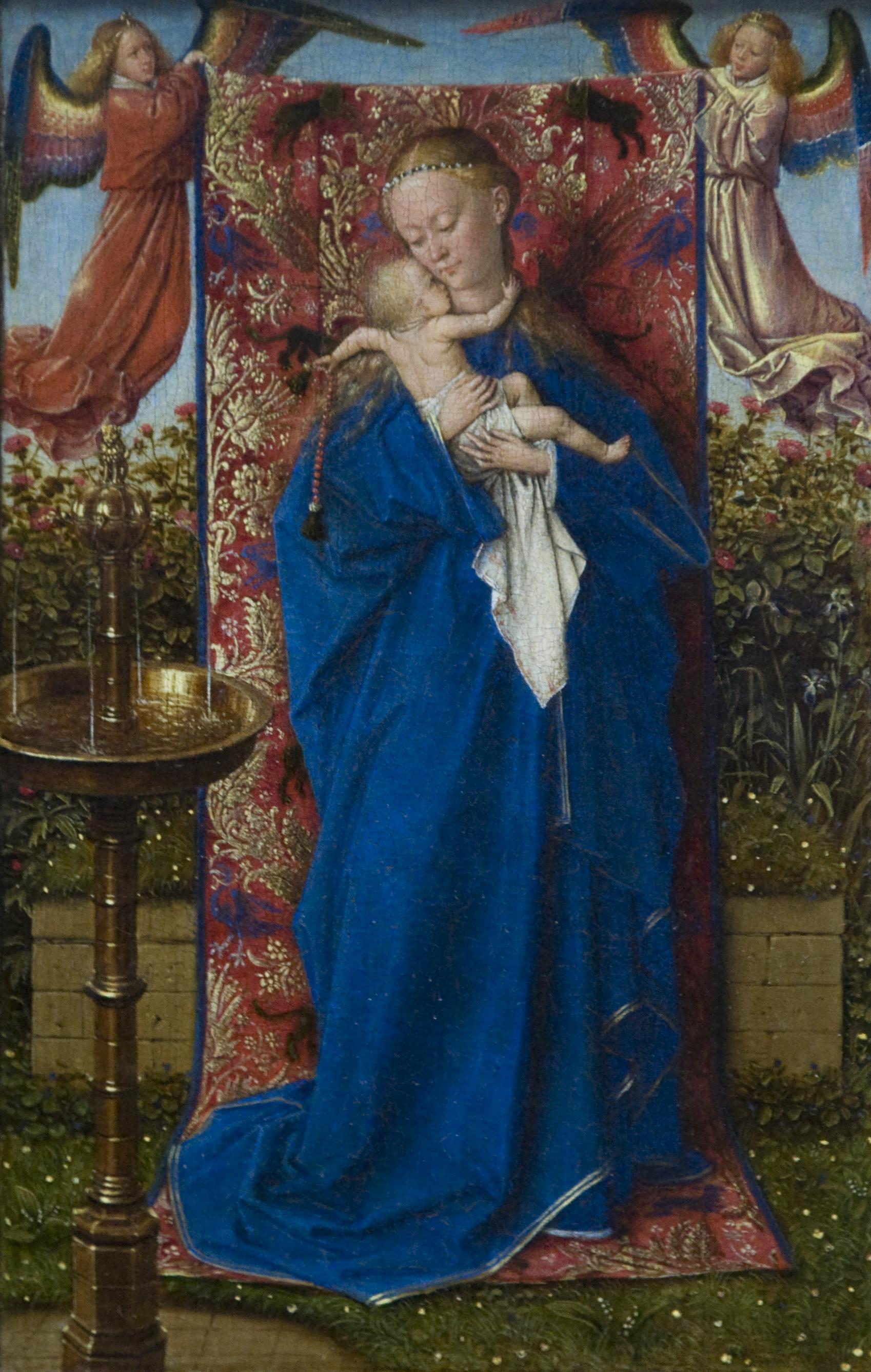The painting depicts a serene outdoor scene under a blue sky with a central focus on a woman and her infant child. The woman, with long blonde hair and a headband-like necklace, is dressed in a large, sapphire-blue robe. She tenderly holds the baby, who is swaddled in a white cloth, and the child clings to her neck. Behind them is a luxurious, red, velvet-like curtain adorned with golden trims and floral patterns, held aloft by two young female angels positioned in the upper left and upper right corners. Each angel, characterized by flowing blonde hair, has rainbow-colored wings; the angel on the left wears a red gown, while the one on the right is dressed in white. The background includes a stone structure partially covered with grass and various flowers, including white blooms and pink rosebuds. To the right of the woman stands a metallic, brownish fountain with a cup of water. The overall scene, rich with earthy and vibrant colors, is bathed in daylight, and the detailed strokes suggest it is a hand-painted artwork.